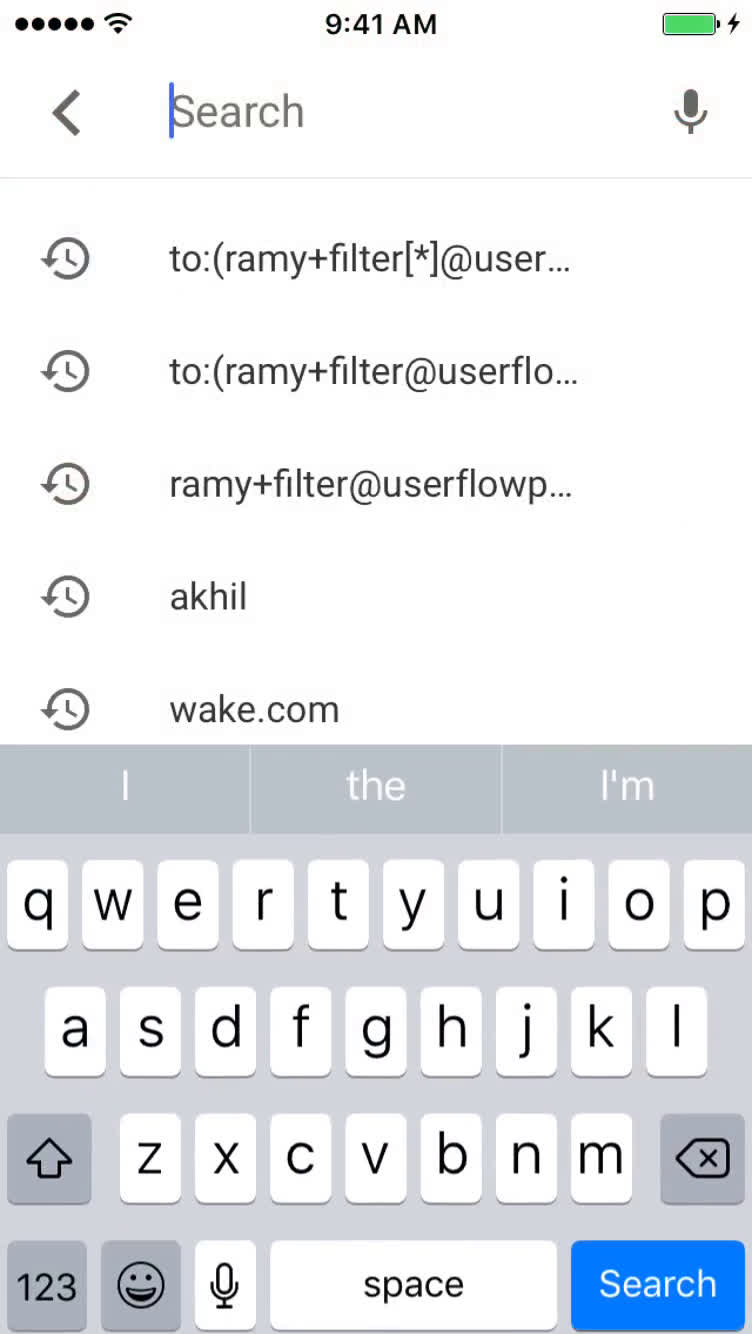This is a detailed screenshot from a phone displaying a search history interface. The top section features a white background with five black dots on the top left, indicating notifications. The current time "9:41 a.m." is displayed centrally at the top, and a full battery icon is situated on the top right.

Below this top bar is a search interface beginning with a left-facing arrow, followed by the word "Search" and a microphone icon. Directly underneath this, in the search history, are multiple entries each accompanied by a circular arrow encasing a clock icon, indicating previously searched items:

1. "To Rammy Plus Filter Star at User..." completes as "To Rammy Plus Filter Star at User dot dot dot."
2. "To Rammy Plus Filter at User F L O..." completes as "To Rammy Plus Filter at User FLO..."
3. "Rammy Plus Filter at User FLOWP..." completes as "Rammy Plus Filter at User FLOWP dot dot dot."
4. "Rammy Plus Filter at User AKHIL."
5. "Wake.com" completes the search history.

Beneath this search history is the phone's keyboard. The keyboard predictions show "I," "the," and "I'm" as selectable options.